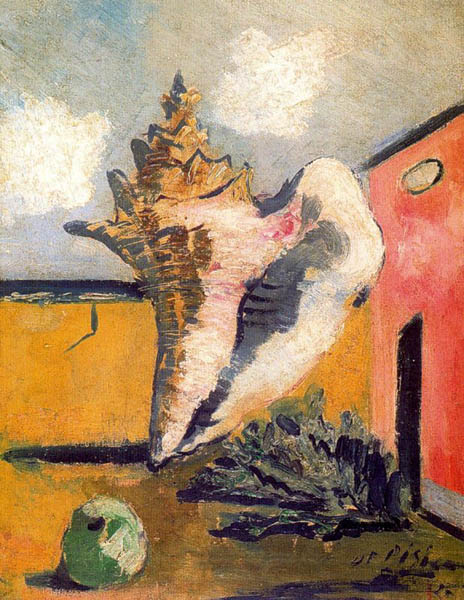This image depicts a surrealist painting featuring a dominant, enormous conch shell with intricate, pointed ends and crown-like top. The shell, predominantly golden-yellow and white with grayish interior, towers over a courtyard area. To the right of the conch shell stands the red-painted front wall of a house with a centrally-placed black rectangular door. The courtyard floor exhibits a vibrant mix of green and yellow hues, dotted with various elements including green bushes, seaweed-like plants, and a circular green object. 

Behind the shell, a cracked, yellow wall extends, juxtaposed against a light blue sky flecked with white clouds. A small tree is visible in the distance on the left side, adding to the surreal and dream-like quality of the scene. The painting appears to be created with oil pastels or paint, and a somewhat indistinct artist's signature is located at the bottom.